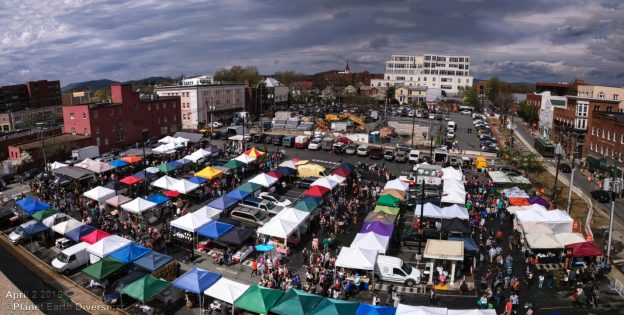The image portrays a bustling outdoor festival set in a city, viewed from an overhead perspective. The central lot is teeming with people and colorful, four-post tents that come together at a singular peak, forming standard booths typically seen at such events. The tents are arranged in neat rows and are vividly colored in shades of white, purple, green, light green, yellow, red, blue, and more. 

In the background and surrounding the festival area, numerous buildings can be seen: red brick buildings to the left, white buildings in the background, and brown brick buildings to the right. The sky above is filled with dark clouds in the center, transitioning to lighter clouds towards the edges.

Towards the top of the image, there is a small roadway bordered by a parking area filled with cars. Additional vehicles are interspersed amongst the tents within the festival lot. A significant white building, resembling a parking garage, is visible in the middle of the image, extending towards the horizon, reinforcing the urban setting of this vibrant gathering.